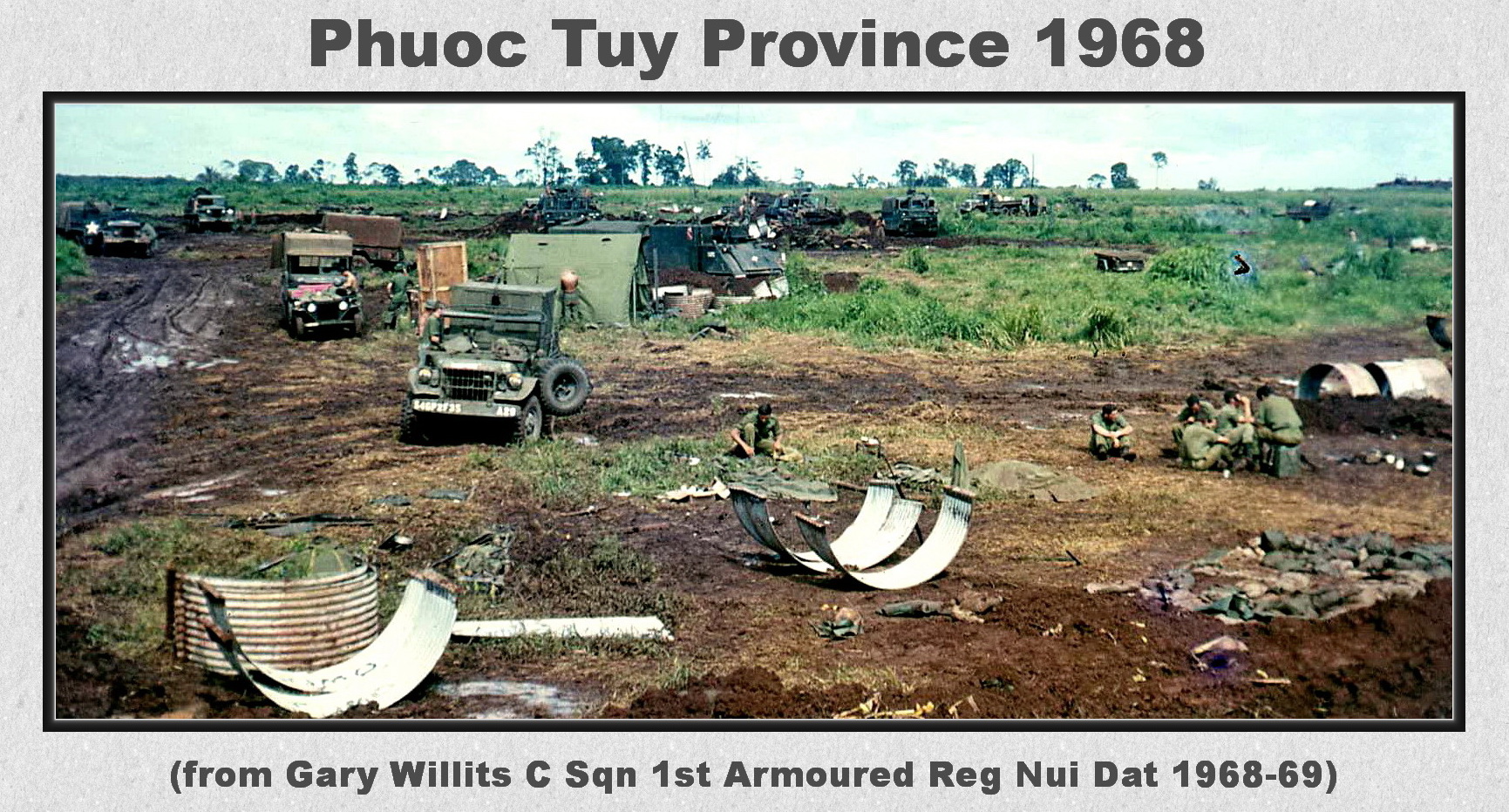The horizontally aligned rectangular picture features a gray and white textured background and a black border around the image. At the top, in black print, it reads "Phuoc Tuy Province, 1968," while the bottom caption states, "From Gary Willits, CSQN, First Armored Reg, Nui Dat, 1968-69." The scene depicts a post-war landscape with a dirt and grassy field, scattered with trees and partially clouded sky. On the left side of the image, military vehicles and pitched tents can be seen amidst the dirt. To the right, a group of soldiers dressed in green uniforms huddle together, with one sitting alone in the center. The ground is littered with broken equipment, including curved metal pieces possibly ripped from a vehicle or weapon. The overall mood of the image reflects the aftermath of a military conflict, possibly the Vietnam War.